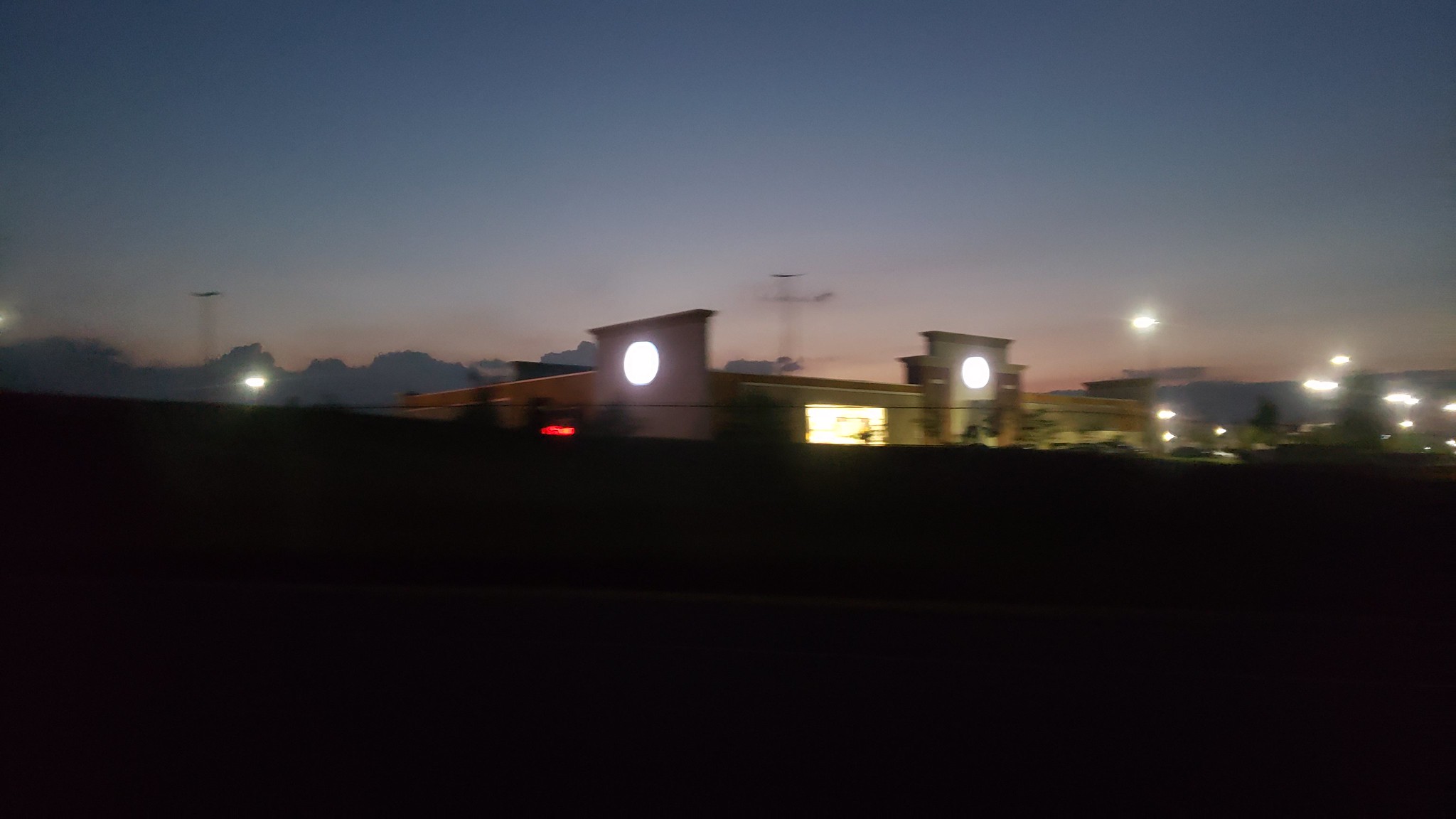This nighttime photograph, likely taken from a moving vehicle, captures a car passing by a brightly lit plaza. The foreground is almost entirely black, suggesting the image was taken through a window or over a barrier. Dominating the center of the image, a shopping center stands with a flat roof and two prominent wall sections that rise higher than the rest of the structure. Each of these sections features a circular light in the middle, while a wide rectangular area of bright yellow light sits between them. The windows of the building emit a brilliant glow, contributing to the overall illumination. Several streetlights are visible, casting additional light on the scene. On the left side of the image, there are trees and electrical poles against a slightly glowing pink horizon, indicating the fading light of dusk or early evening. The right side of the picture shows a concentration of lights, possibly from other buildings or streetlights. The image conveys a sense of motion and the ambiance of a bustling, illuminated plaza at night.